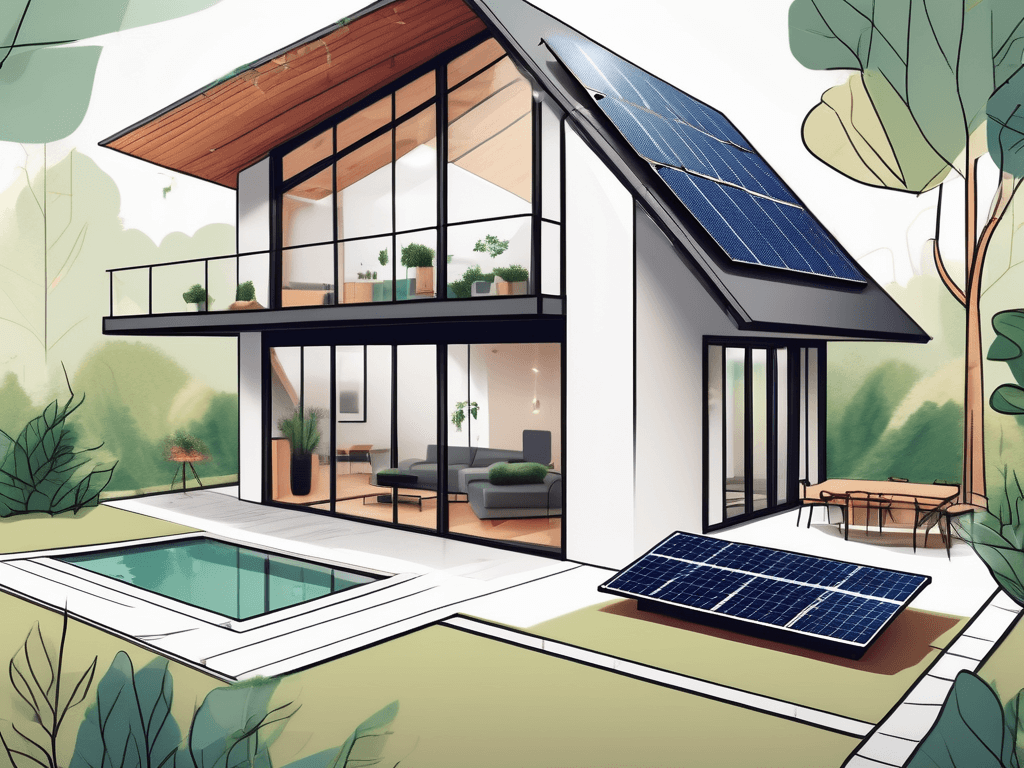The image depicts a detailed, digital illustration of a modern, two-story house with sleek white walls and expansive glass windows that stretch from top to bottom. The house features a balcony with a black wrought-iron railing on the upper level, allowing views of the interior, which includes sofas, chairs, and potted plants. The ground level reveals wooden floors and a gray couch visible through the glass facade. Both the roof and the garden in the lower right corner are equipped with large solar panels. Adjacent to the house is a small rectangular pool, surrounded by various trees with brown trunks and green foliage, and a yard furnished with a table, benches, and chairs. The scene is further enriched with green and white vegetation, emphasizing its artful, almost cartoony style.